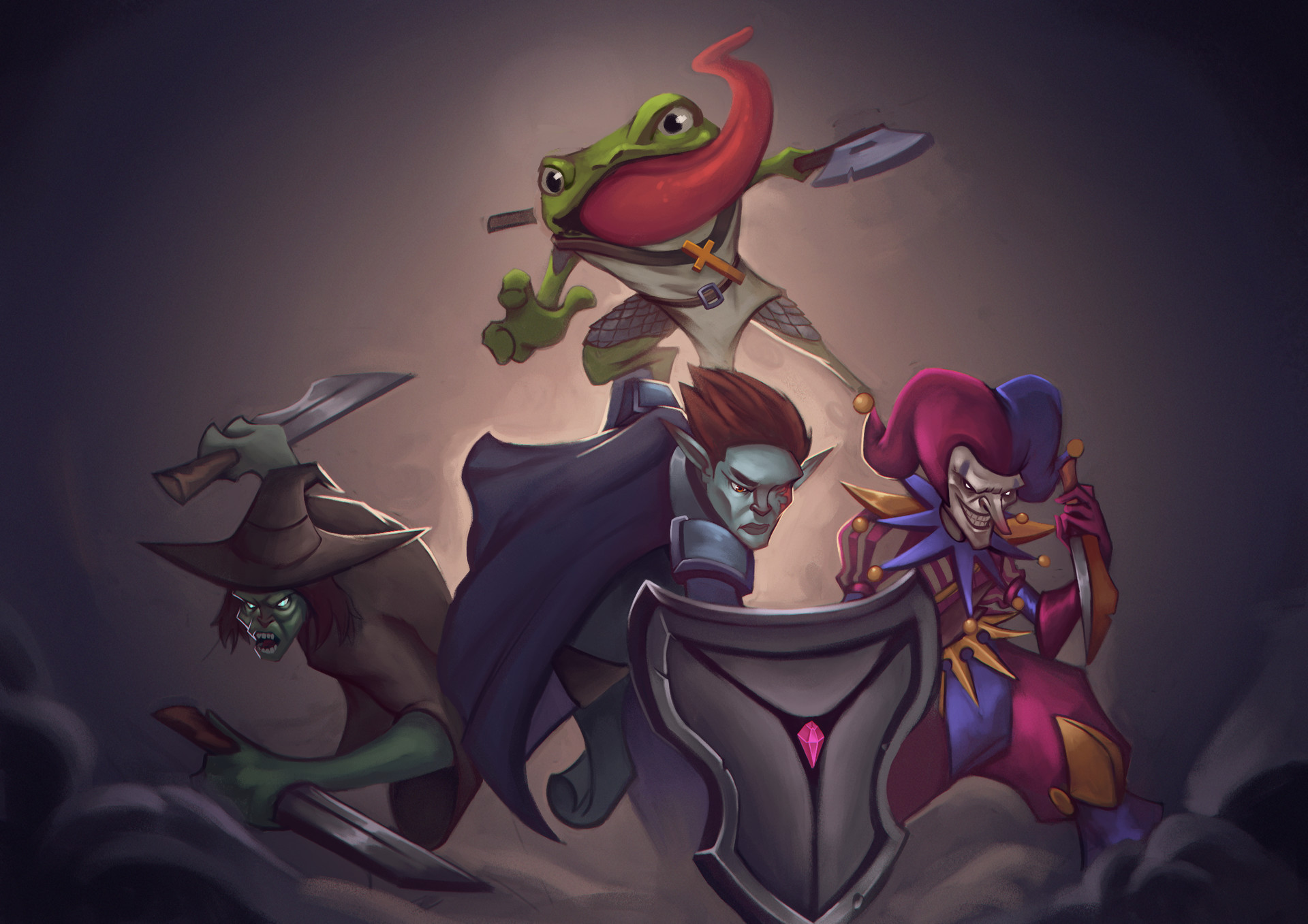The image is a highly detailed digital illustration of cartoon characters in a game-like setting, featuring a dark, fantastical theme. At the center is a gargoyle-like character with a green face, long pointy ears, and red hair, wielding a shield adorned with a pink gem angled defensively. To his left stands a warrior resembling a witch, with green skin, garbed in a brown witch's hat and coat, and holding a knife in each hand. On the right is a sinister jester-like character with a billowy blue and red hat, pointed collar, and a knife ready in his right hand. Above all of them, a giant frog fighter with a green face, a protruding red tongue, and a beige smock sporting a brown cross, wields an axe menacingly. This dynamic group is set against a backdrop that transitions from bright to progressively dark hues, with purple tinges in the corners and cloud-like formations at the bottom, enhancing the eerie ambiance.